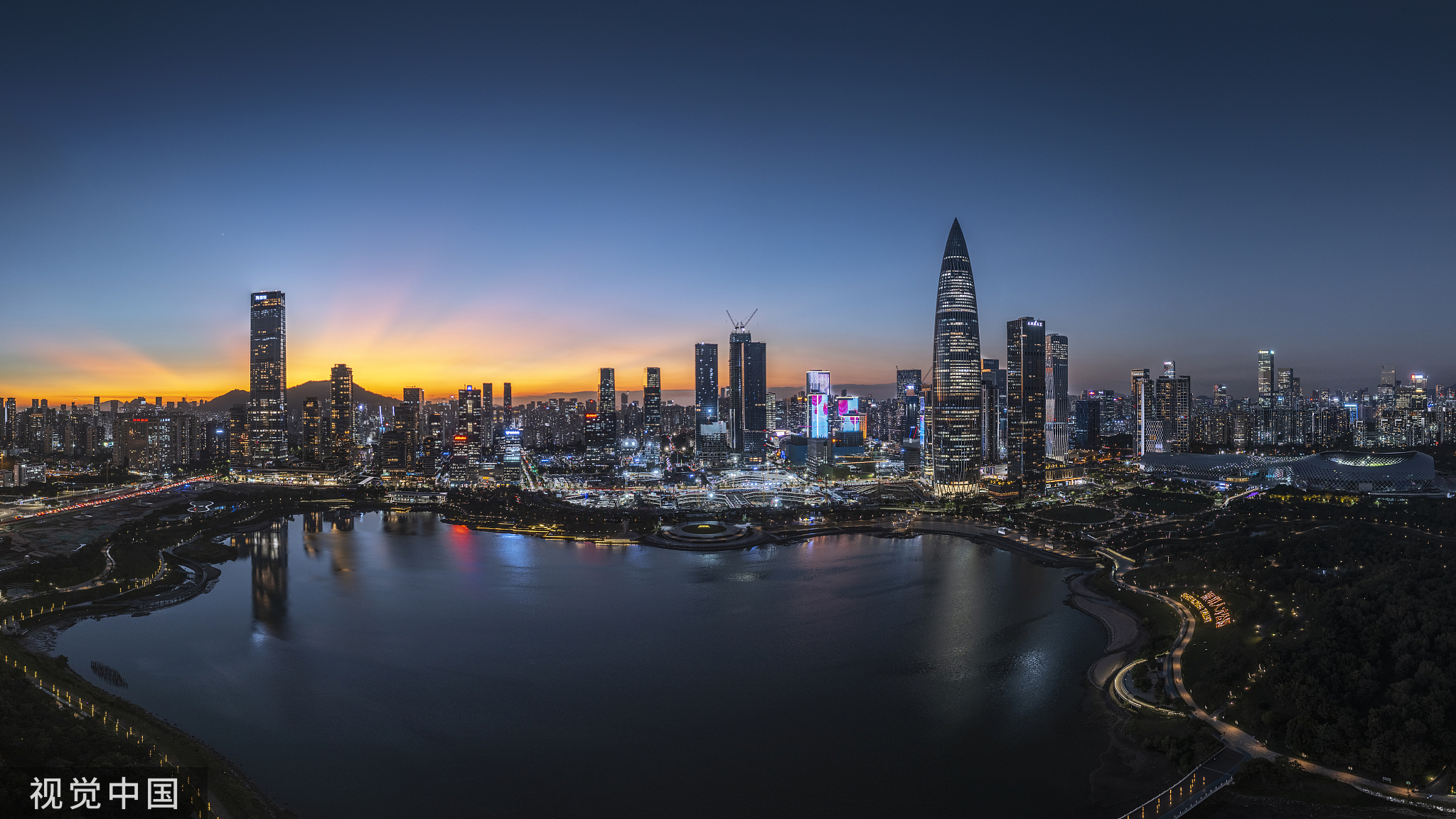The image captures a professional, stunning cityscape of a vast urban area near a beautifully curbed harbor. It appears to be taken from a high vantage point, showcasing the city at twilight, just as the sun is setting or has recently set. The sky transitions from bright hues of yellow, orange, and pink near the horizon to a darker grayish blue as it ascends, with high, streaky white clouds adding texture to the scene. The harbor’s calm water reflects the myriad lights of a sprawling and densely built city, giving an almost magical shimmer to the entire scene.

To the left, a section of the image features a series of Chinese characters, indicating the likely location within mainland China. The harbor curves gently, bordered by lighted roadways, which highlight the peninsula on the right side dotted with trees and street lights. An elegant bridge arches over the water on the right, enhancing the architectural beauty of the city.

Numerous skyscrapers dominate the skyline, their windows ablaze with light, creating a striking contrast against the twilight sky. In the far distance, vibrant billboards and illuminated signs—colored blue and red—add a contemporary urban touch. The towering buildings, some more than two dozen in height, grow smaller toward the left, maintaining a consistent flow of lights that guide the eye around the expanse of the harbor.

The entirety of this scene is brought together by the harmonious blend of natural dawn light and urban luminosity, painting the picture of a bustling, cosmopolitan area transitioning from day to night.